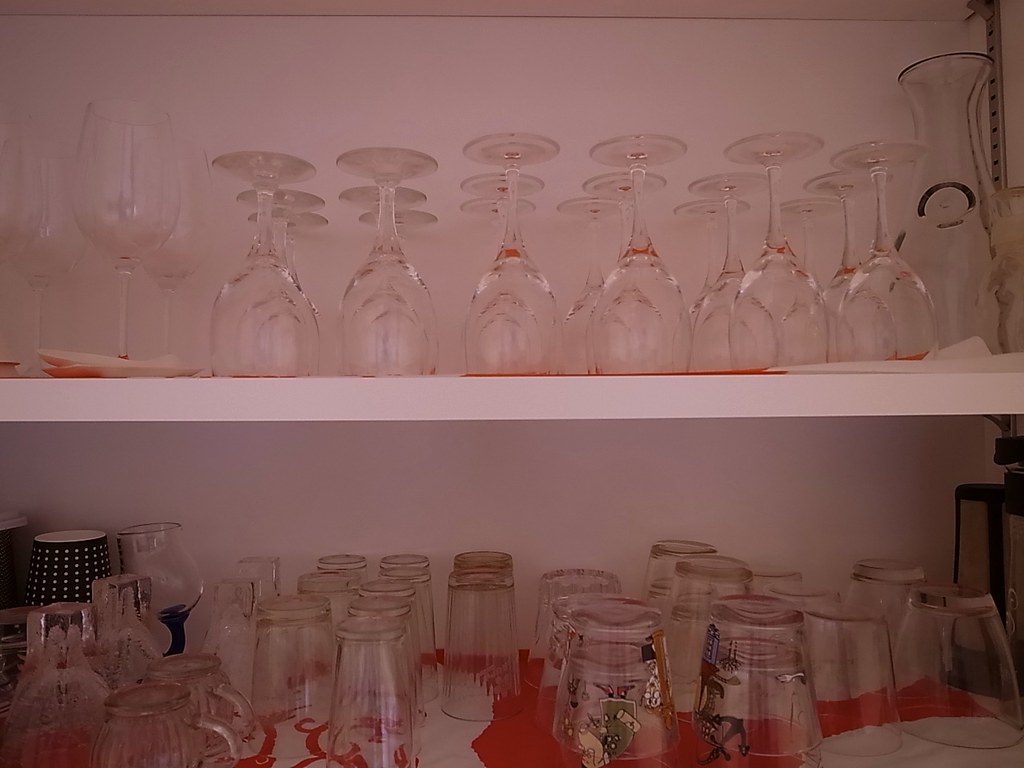The image depicts a two-shelf cabinet adorned with a red and white patterned liner, holding a variety of glassware. On the top shelf, there are several goblets and wine glasses, some standing upright while others are stacked upside down on their lips. To the right, a glass vase is visible. The bottom shelf features simpler glassware: small tea cups, coffee mugs, and standard drinking glasses, all positioned upside down. The cabinet itself appears to be pink, with the top shelf lined with goblets on the left standing on their bases, transitioning to inverted glasses toward the center. The bottom shelf's left side hosts mugs and tea cups, while the rest of the shelf displays an assortment of decorated and plain glasses. A distinct black and white polka-dotted coffee mug is also noted on the bottom shelf.